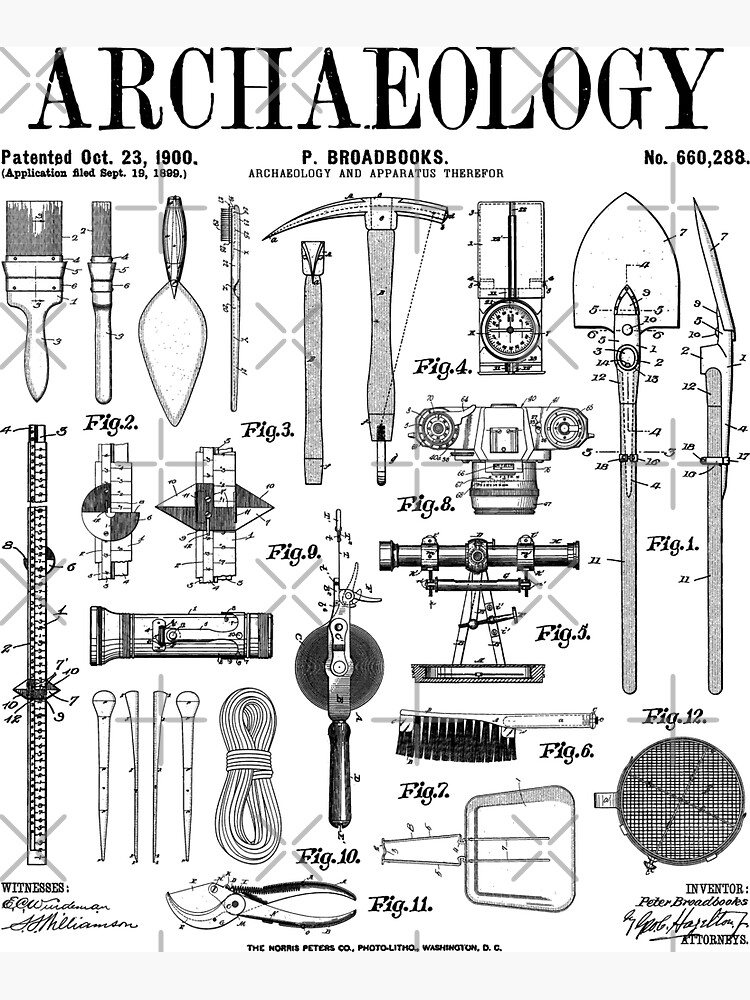This detailed black-and-white drawing, resembling a magazine cover or a brochure, prominently features the bold title "ARCHAEOLOGY" at the top. The text, almost appearing as a headline and byline, indicates a patent date of October 23, 1900, for "P. Broadbeck's Archaeology and Apparatus," with patent number 660,288. The image showcases a variety of archaeological tools meticulously sketched with specific measurements and pointed details, suggesting their use in fieldwork.

The tools depicted include a paintbrush and trowel for brushing off artifacts, a small brush similar to a toothbrush, a pick, and a foldable shovel akin to military equipment. Other instruments include a compass, a sifter, a pair of pliers, and a wire brush. Distinct figures also represent a camera, possibly an SLR type, a jack for elevation adjustments, a rope tied in a specific knot, and a grate for sifting materials. Additional tools such as chisels and a flashlight are also illustrated, offering a comprehensive view of the essential apparatus used in archaeology as of the early 20th century.